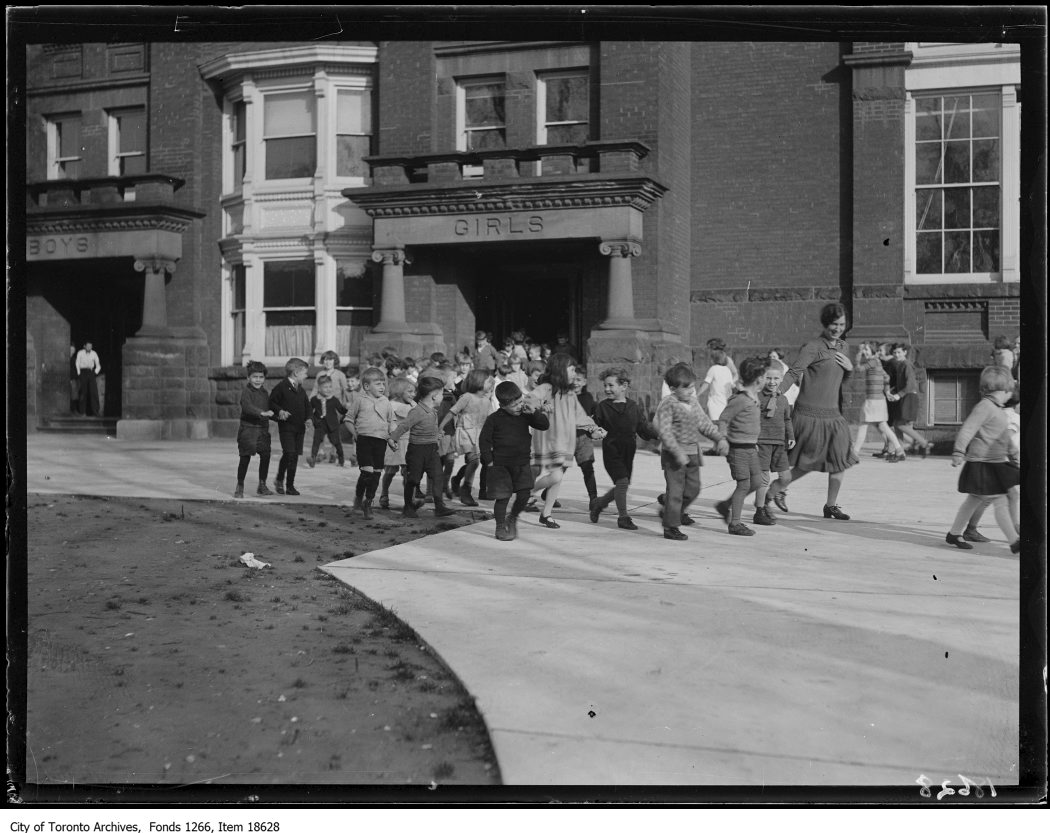This vintage black-and-white photograph, labeled "City of Toronto Archives Fonds 1266, Item 18628" in the lower left corner, captures a scene from the 1930s or 1940s in front of a masonry brick school building, potentially located in a big city like Toronto. The structure features prominent, chiseled stone entrances with the words "Boys" on the left and "Girls" on the right, each flanked by pillars and topped with a pediment. A group of young children, likely kindergarten-aged, dressed in period attire including high knee socks, shorts, and sweaters, are happily holding hands as they walk across the pavement, seemingly led by a female teacher. The children, smiling and appearing to be on a field trip or simply enjoying a break, move in rows of three from the "Girls" entrance toward the right of the frame. Two men stand near the "Boys" entrance, further highlighting the gender-segregated design of the era. The image is bordered by a black frame, indicating it is a print made from a film negative, and some indistinct white numbers are visible in reverse at the lower right corner of the photograph.